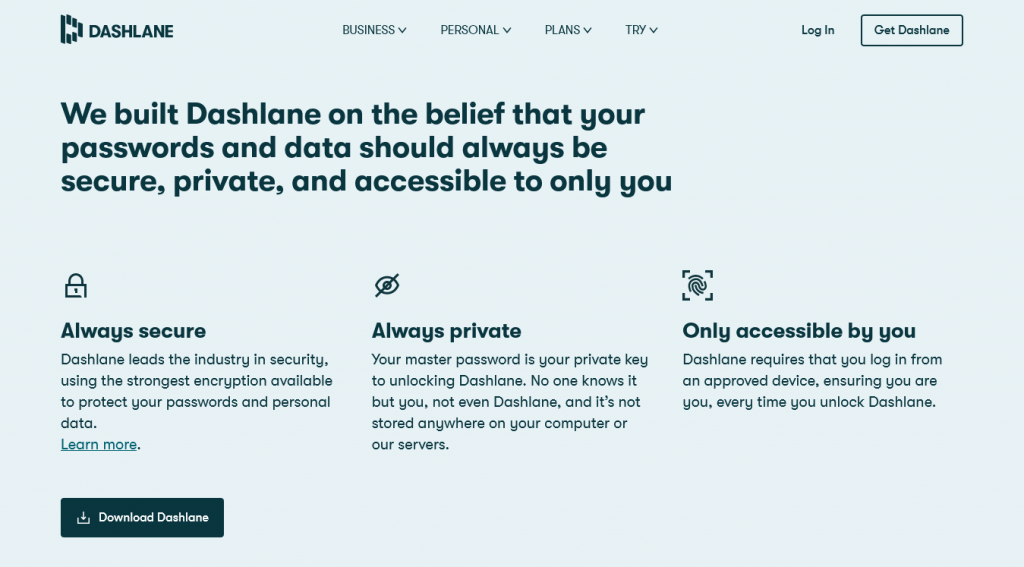A light blue, horizontal rectangular box features prominently with all print in black. In the top left corner, it reads "Dashlane" alongside the Dashlane logo. Across the top are categories labeled "Business" (with a drop-down arrow), "Personal" (drop-down arrow), "Plans" (drop-down arrow), and "Try" (drop-down arrow). On the far right, it offers "Login" and a "Get Dashlane" button outlined in black.

In bold, black text, a statement reads: "We built Dashlane on the belief that your passwords and data should always be secure, private, and accessible to only you."

Beneath this statement, three horizontally arranged sections highlight key service features:

1. **Always Secure**:
   - Accompanied by a padlock icon.
   - Caption: "Dashlane leads the industry in security, using the strongest encryption available to protect your passwords and personal data. Learn more."
   - A black "Download Dashlane" button is situated below this description.

2. **Always Private**:
   - Accompanied by an icon of an "I" with a line through it.
   - Caption: "Your master password is your private key to unlocking Dashlane. No one knows it but you, not even Dashlane, and it's not stored anywhere on your computer or our servers."

3. **Only Accessible by You**:
   - Accompanied by a QR code icon.
   - Caption: "Dashlane requires that you log in from an approved device, ensuring you are you every time you unlock Dashlane."